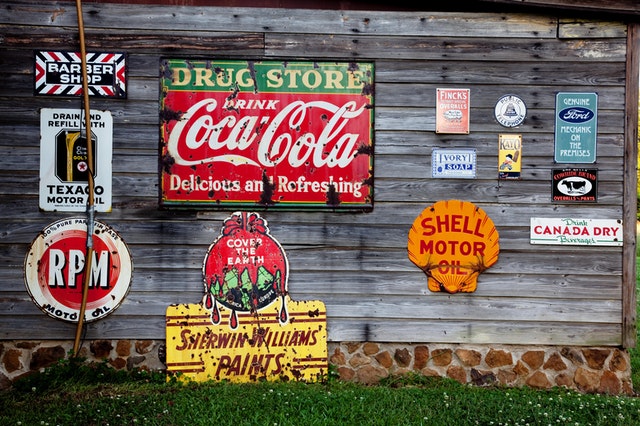This image captures the side of a vintage, rustic building, possibly a barn or an old shack, showcasing a fascinating collage of retro signs affixed to its wooden plank siding, which is set above a stone foundation. Dominating the scene is an array of weathered signs, each telling a piece of history. Prominently, there's a large, rusted red rectangular sign proclaiming "Drug Store, Drink Coca-Cola, Delicious & Refreshing," standing out among the collection. To its right, a yellow sign with a seashell icon reads "Shell Motor Oil," and beneath it, another yellow sign with red lettering advertises "Cover the Earth, Sherwin-Williams Paints." Additional signs include "Drink Canada Dry Beverages," "Barbershop," "RPM," "Texaco Motor Oil," and "Genuine Ford Mechanic on the Premises." Smaller, less legible signs pepper the structure, adding to the nostalgic ambiance. The ground below is covered with grass, complementing the overall aged and rustic charm of the scene.